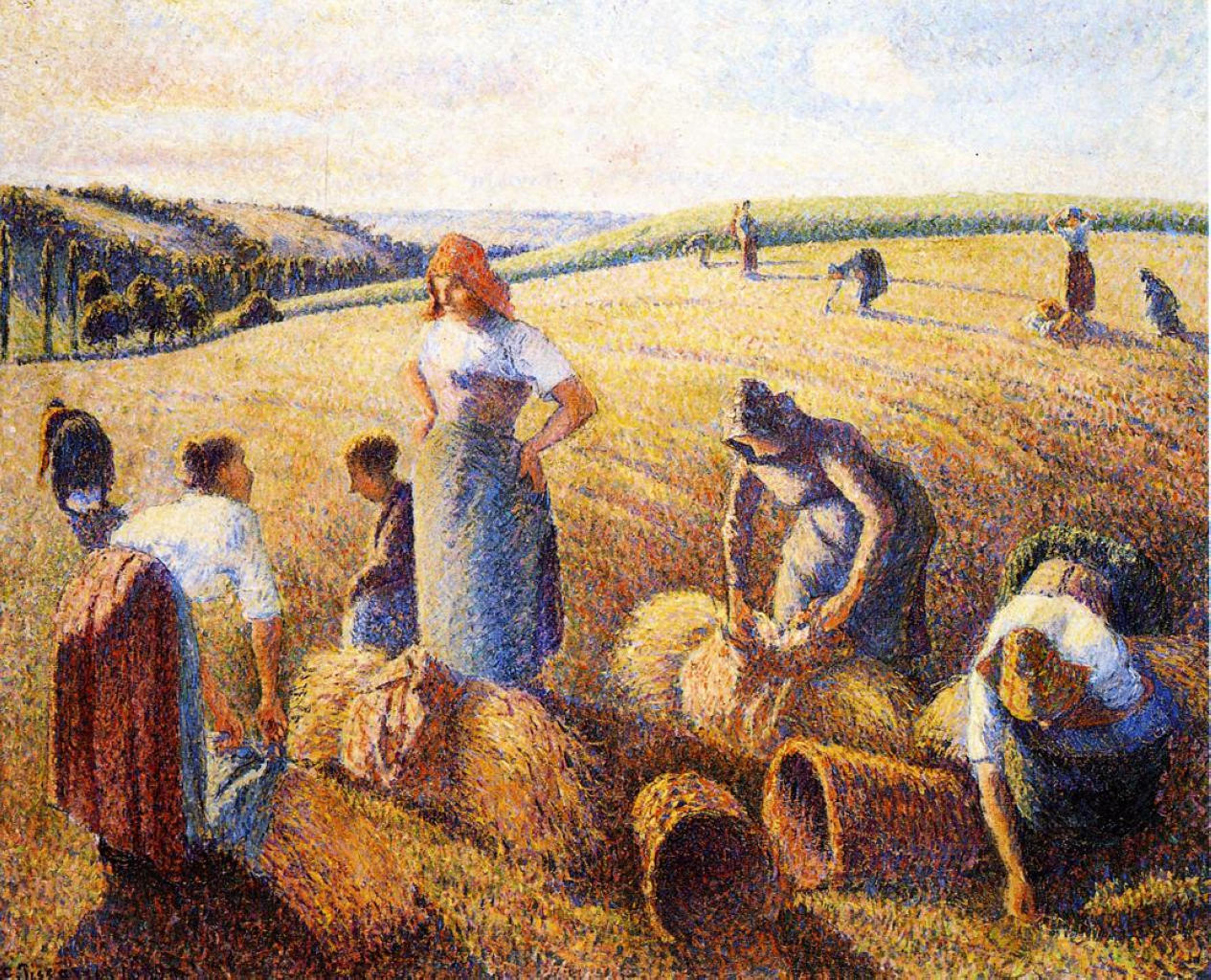This impressionistic painting, reminiscent of Van Gogh's style with its short, textural brush strokes, portrays a bustling medieval hayfield scene. The composition captures a group of farmers, primarily women, dressed in traditional full-length skirts and handkerchiefs, diligently working amidst the rolling yellow and green hills. In the foreground, a tall woman in an orange bandana, white shirt, and blue skirt stands prominently, conversing sternly with a shorter, more robust woman who is bent over, maybe under her direction. Nearby, a woman in a gray hooded robe ties up straw or hay. Surrounding them are other women busy wrapping hay or wheat into baskets for transport, while a line of women in the background are seen bending over, either harvesting or planting seeds. To the left, the scene is bordered by bushes and distant trees, and to the right, the landscape opens into more vegetation. Above, the sky transitions from a white-blue to an orange hue on the left, hinting at the sun. The overall color palette is dominated by the yellowish-beige of the wheat, contributing to the vivid and dynamic portrayal of rural life.